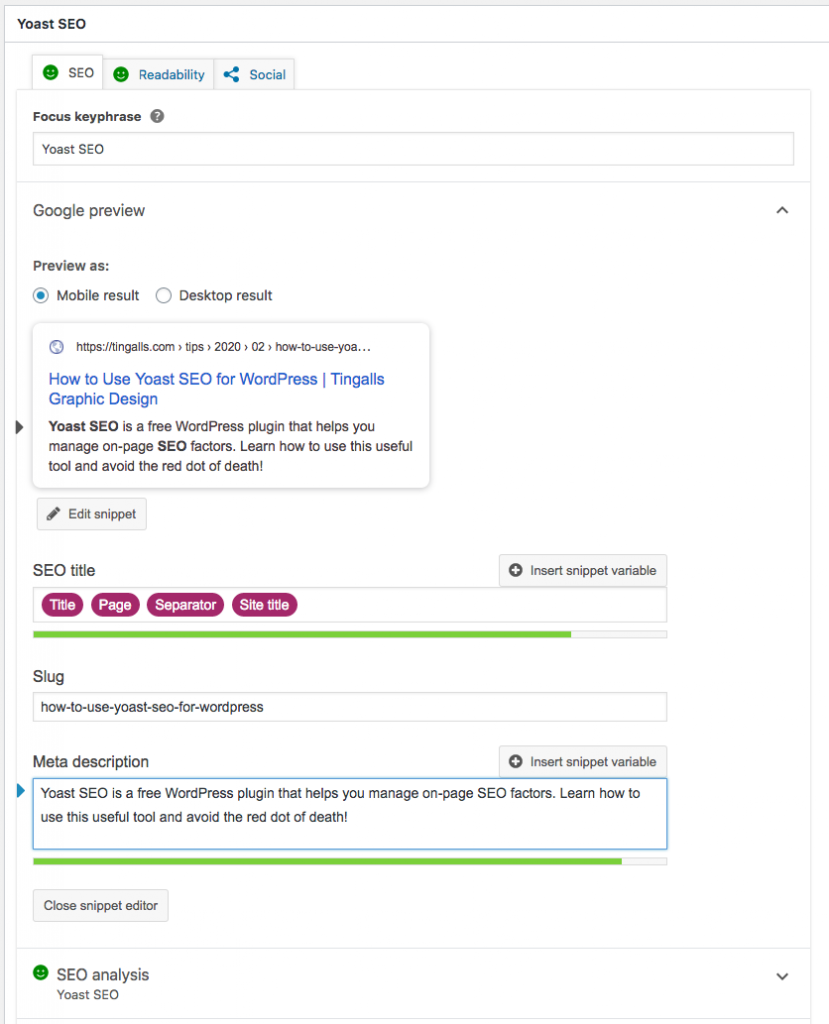In this image, a screenshot of the Yoast SEO plugin interface is displayed. In the upper left corner, the Yoast SEO logo is visible. Below the logo, there are three tabs: SEO, Readability, and Social. The SEO tab appears to be selected. Under this tab, there's a section labeled "Focus Keyphrase" with a text box containing the phrase "Yoast SEO."

Beneath the Focus Keyphrase section, there is a "Google Preview" area, allowing users to preview their content as it would appear in Google search results, with options to view as a mobile or desktop result. The mobile result option is currently selected, showing a preview listing titled "How to Use Yoast SEO for WordPress" from 10 Gals Graphic Design.

Below the preview, there's a section for editing the SEO title, slug, and meta description. The meta description text box contains two sentences. At the bottom left of the section, there's a button labeled "Close Snippet Editor."

This detailed interface allows users to optimize their content for search engines directly within WordPress by managing focus keyphrases and previewing search result appearances.